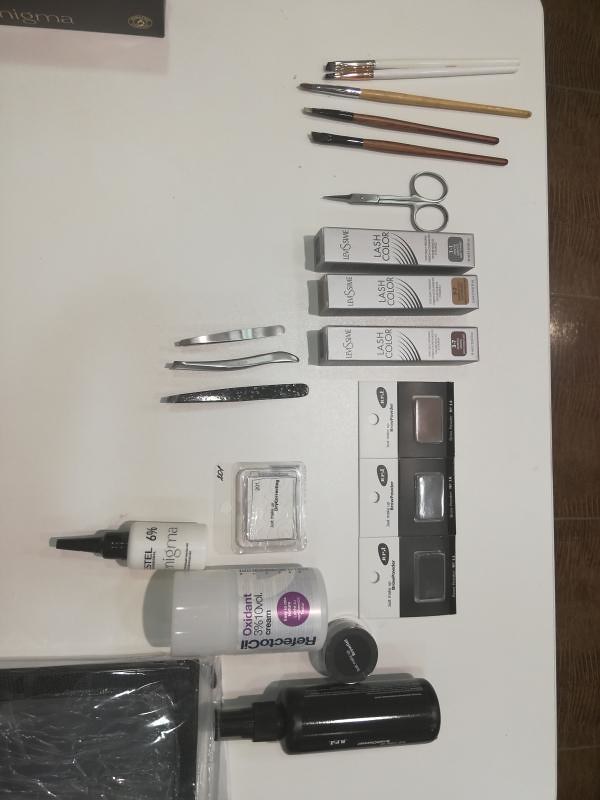Indoor color photograph depicting a white countertop arrayed with various manicure and makeup tools. From left to right, the scene is meticulously organized with both functional and grooming items.

In the bottom left corner, a shiny black bag captures light. Positioned horizontally to its right is a black bottle equipped with a spray cap angled to the left. Just above this bottle sits a small jar with a black cap. Slightly higher and to the left of the jar is a cylindrical container adorned with a white label, featuring text that states "Oxidant 3%" and additional unreadable text.

Further above and to the left is another small bottle with a tall, thin black cap, oriented to the left. This bottle’s label reads "6%" and "NIGMA." Centrally positioned in the frame is a small silver square pack.

In the middle of the image, three different styled tweezers are lined up horizontally with their tips pointed to the left. Two are stainless steel, while one appears to be painted black.

Shifting our focus to the upper right corner and moving downward, a column of items begins with two short-bristled brushes featuring white handles. Below these, a longer-handled wooden brush with a silver tip is placed. Further down, two identical shorter brushes with brown handles are aligned. Next, a pair of small shears, likely intended for trimming eyebrow or eyelash hairs, is visible.

Near the lower right corner, three silver boxes labeled "lash color" are arranged horizontally. Finally, situated below these boxes are three rectangular packets, presumably containing eyelashes. Each packet has a clear window on the right, though no legible text is evident.